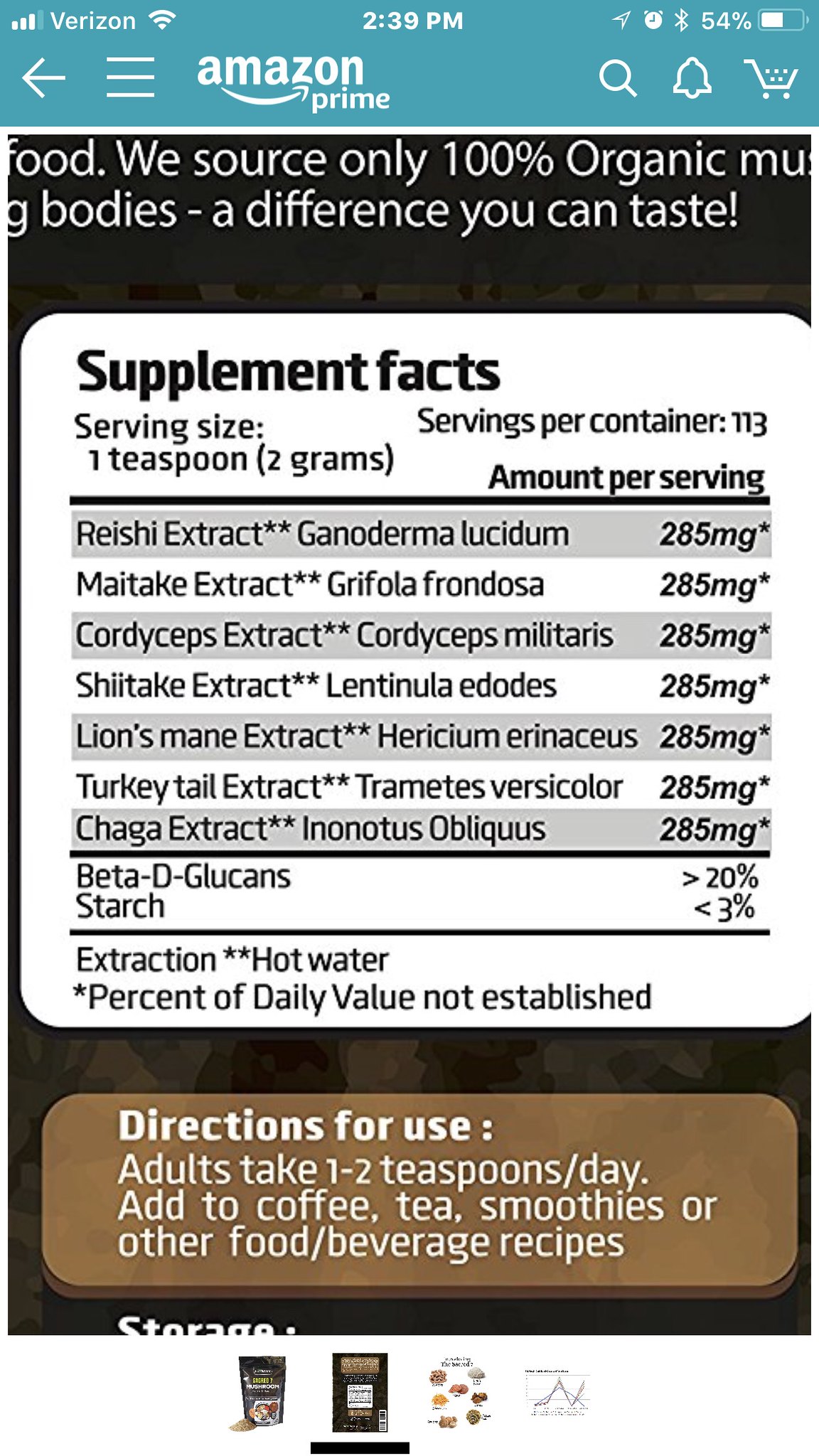This close-up image showcases the details from the product page of a dietary supplement on Amazon Prime. The focus is on the supplement facts panel of a large container with 113 servings, where each serving is just one teaspoon. The supplement contains a blend of various mushroom extracts, including Reishi, Maitake, Cordyceps, Shiitake, Lion's Mane, and Turkey Tail Extract. These extracts are obtained through a hot water extraction process. Notably, the product lacks an established daily value for some of the ingredients. Instructions recommend taking one to two teaspoons daily, mixed into coffee, tea, smoothies, or other beverages. At the bottom of the image, there are smaller pictures showing the product's packaging and potentially its benefits, although the exact nature of the supplement remains unspecified.